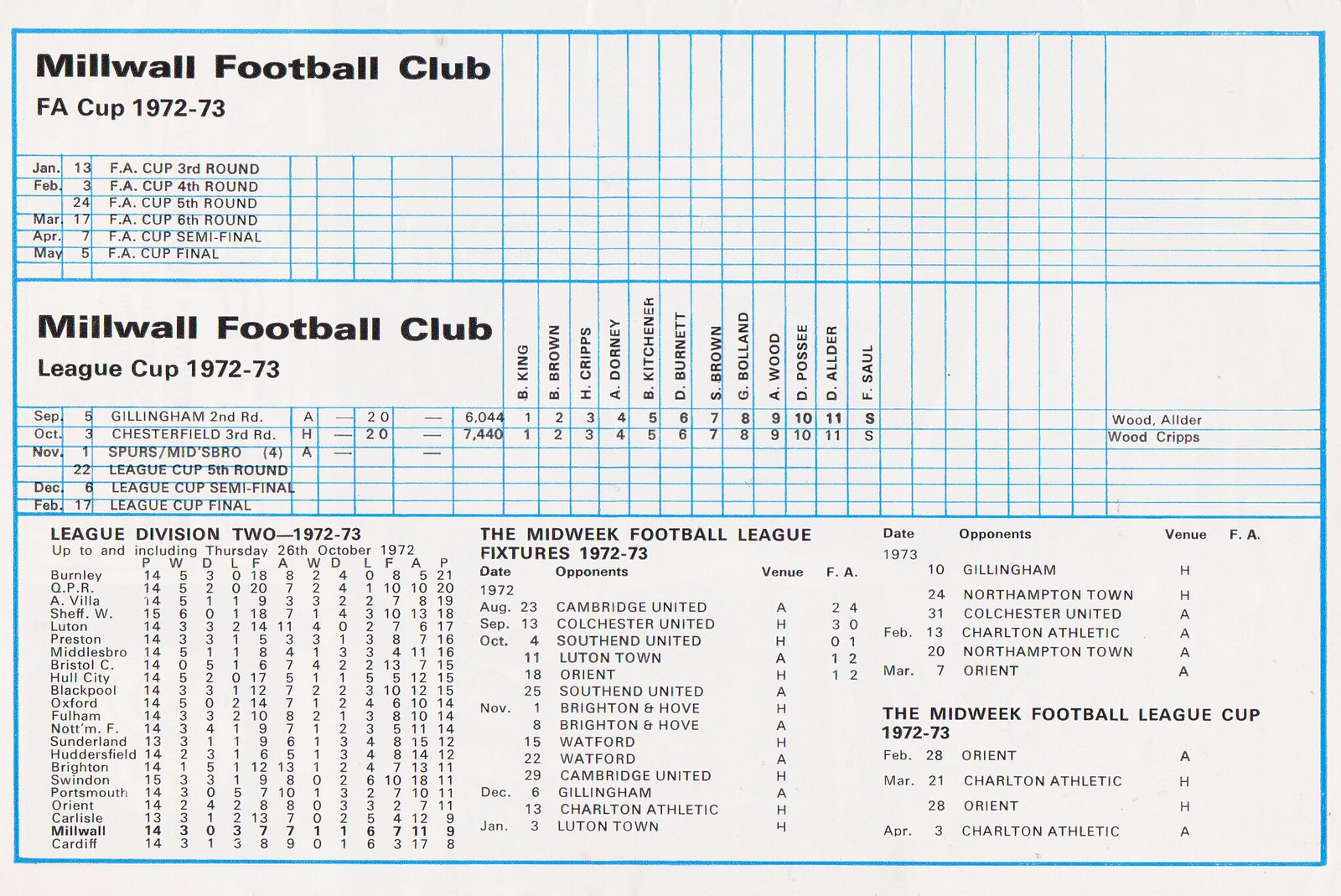An informational sheet, set on off-white paper with a light blue border, details the Millwall Football Club's activities for the 1972-73 season. The sheet is divided into three main sections. 

At the top, the title "Millwall Football Club" is prominently displayed, followed by "F.A. Cup 1972-73." This section contains a blue-lined grid listing months from January to May along with match dates and brief descriptions of the rounds, such as the third round through to the final.

The middle section, under "Millwall Football Club League Cup 1972-73," similarly details the club's League Cup fixtures with dates and points assigned to players alongside their names. This period covers from September through to December, structured again in a blue-lined grid format.

The bottom third contains three distinct columns providing additional information: "League Division II 1972-73" featuring a list of player names and their corresponding statistics; "Midweek Football League fixtures 1972-73," and "Midweek Football League Cup 1972-73," both extending to fill the remaining part of the page. Each section is meticulously organized in a grid, presenting dates, fixtures, and player-related data.